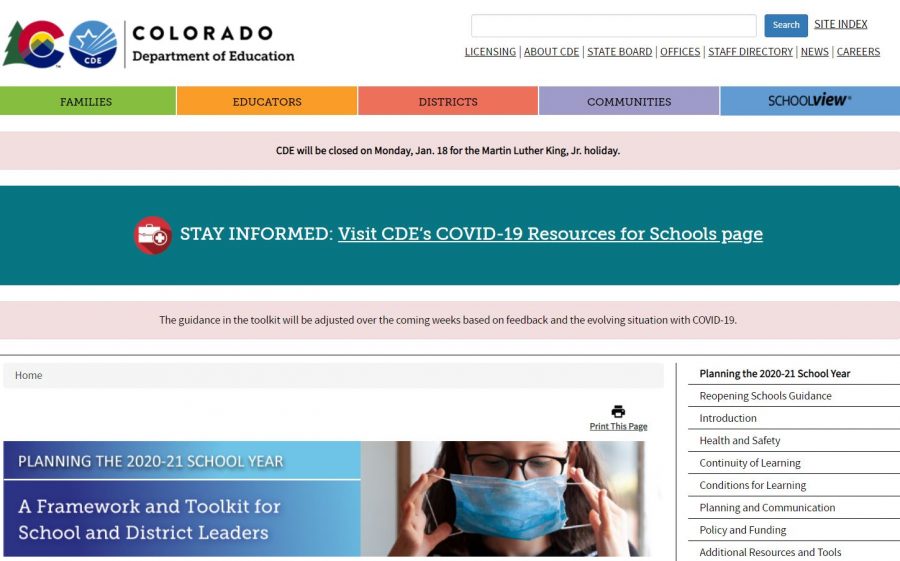The screen capture depicts the Colorado Department of Education (CDE) website. At the top left, the CDE logo features a pine tree, the letter "C" symbolizing Colorado, and mountains, accompanied by a star beam design signifying the department. Adjacent to the logos, clear text reads "Colorado Department of Education."

The top navigation bar includes a search bar and links labeled "Site Index," "Licensing," "About CDE," "State Board," "Offices," "Staff Directory," "News," and "Careers." Below this, category buttons for "Families," "Educators," "Districts," "Communities," and "School View" enable easy navigation.

A notification bar with a teal background at the top of the page warns that the CDE will be closed on Monday, January 18th, in observance of the Martin Luther King Jr. holiday. Another message encourages users to stay informed by visiting CDE's COVID-19 resources for schools, noting that the guidance and toolkit will be updated based on feedback and the evolving COVID-19 situation.

The header image features a child wearing a mask, with accompanying text that reads "Planning for the 2020-2021 School Year." This section provides a framework and toolkit for school and district leaders. On the right side of this segment, various buttons and text links offer further resources and information.